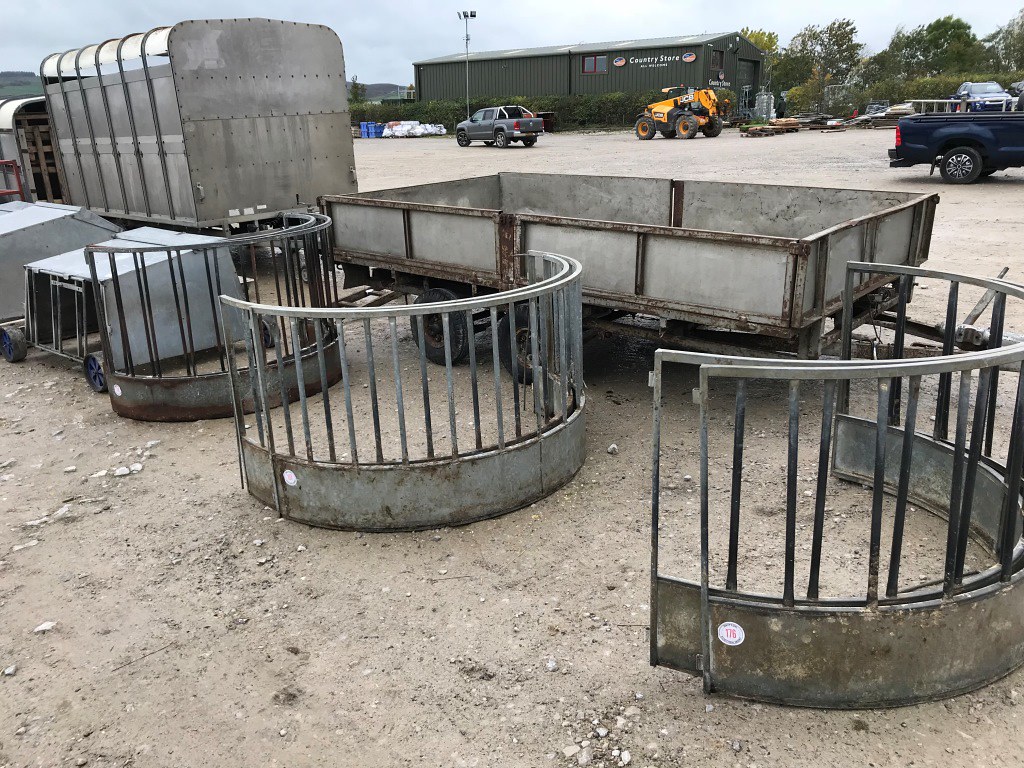The photograph captures an outdoor storage area, possibly part of a country store's parking lot, filled with various rusted metal equipment. Dominating the foreground are three half-circle metal structures with bars; the first has widely spaced bars, the second has bars that are closer together, and the third also has bars but appears very worn and rusted. Nearby, there's a large metal storage trailer with solid walls and a solid top, mounted on wheels, that looks somewhat like it could transport animals but isn't intended for that purpose. The trailer, very degraded with rust inside and outside, sits alongside an open storage container with a lid, partially buried in the dirt. In the distant background, a couple of trucks and a tractor are visible near a large industrial-size brown building with "Country Store" emblazoned on it, flanked by American flag emblems. The setting is a gravel and dirt surface, suggesting a rustic, utilitarian outdoor environment conducive for agricultural or storage use.